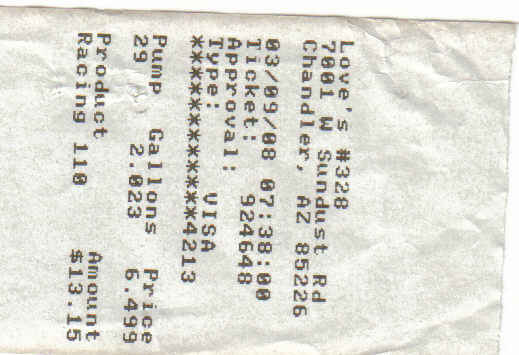This image features a scanned, grainy receipt with a slightly serrated, yet straight, edge on the right-hand side. The receipt is oriented sideways at a 90-degree angle, requiring it to be read from left to right. The text begins with "Love's No. 3287001, West Sundust Road." Below this, the date and time of the transaction, along with the approval details, are listed. A Visa card, identifiable by the type and the partial number "4213," was used. The transaction specifics include "Pump 29," "Gallons: 20.23," and a per-gallon price of $6.499. The total amount charged is $131.50. This receipt documents a fuel purchase at an unusually high price per gallon, potentially explaining the significance of retaining it.